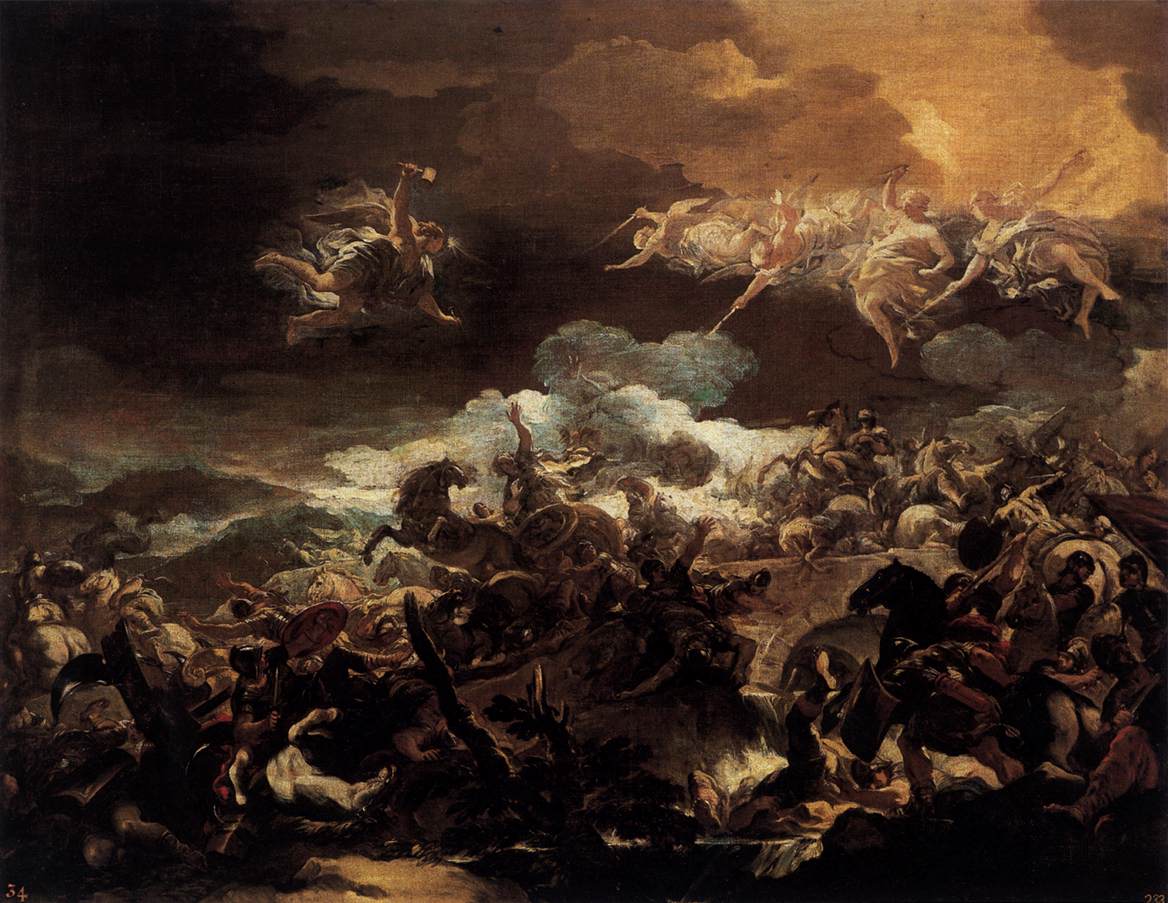The image is a dramatic and detailed painting, possibly watercolor or oil, depicting an intense war scene from what seems to be the 16th or 17th century. The central focus is on the battle between two armies equipped with swords and sabers, many of whom are on horseback, engaged in combat and possibly crossing a bridge. Below, the ground is teeming with dozens of soldiers dressed in armor, with horses amidst the chaos, emphasizing the sheer magnitude of the conflict.

Above the fray, the sky is dark and ominous, streaked with clouds and a rare glimmer of sunlight breaking through in the upper right corner. There is a mystical dimension added by the presence of several beings that appear to be angels or gods. These figures, numbering around five, are semi-clothed in white linens and float above the battlefield. One of these celestial beings on the center left appears to be holding a hammer, poised as though to strike or intervene, while others point downward, possibly awaiting the souls of fallen soldiers. The entire scene has a dark tone, almost as if occurring at night, punctuated by the stark whiteness of the clouds and the linen garments of the angels. Notably, there is a number "34" inscribed in the bottom left-hand corner of the painting, adding a touch of mystery to its identity and origin.